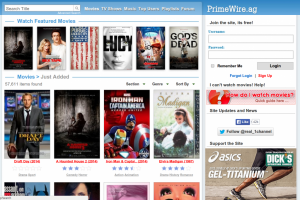On the Prime Wire homepage, the layout features a search bar on the left-hand side where users can input a movie title to find specific content. The text within the search bar is somewhat hard to read, but it indicates that you should search by "title." Below this, there are sections labeled "Movies," "TVs," and some blurred options, followed by "Playlists" and another blurred label. 

Beneath these headings, the page showcases a section titled "Watch Featured Movies," displaying six movie posters. Further down, a blue heading labeled "Movies, Just Added" presents four newly added movies in a larger format, with partial previews of four additional movies below them.

On the right-hand side, the Prime Wire interface includes a login section with fields for Username and Password, along with options for "Login," "Remember Me," "Forgot Login," and "Sign Up." There are also assistance links such as "I Can't Watch My Movies," "Help," and "How Do I Watch Movies." Supporting the site is an advertisement for "Ozak Gel Titanium by Dix," displayed at the bottom of the login section.